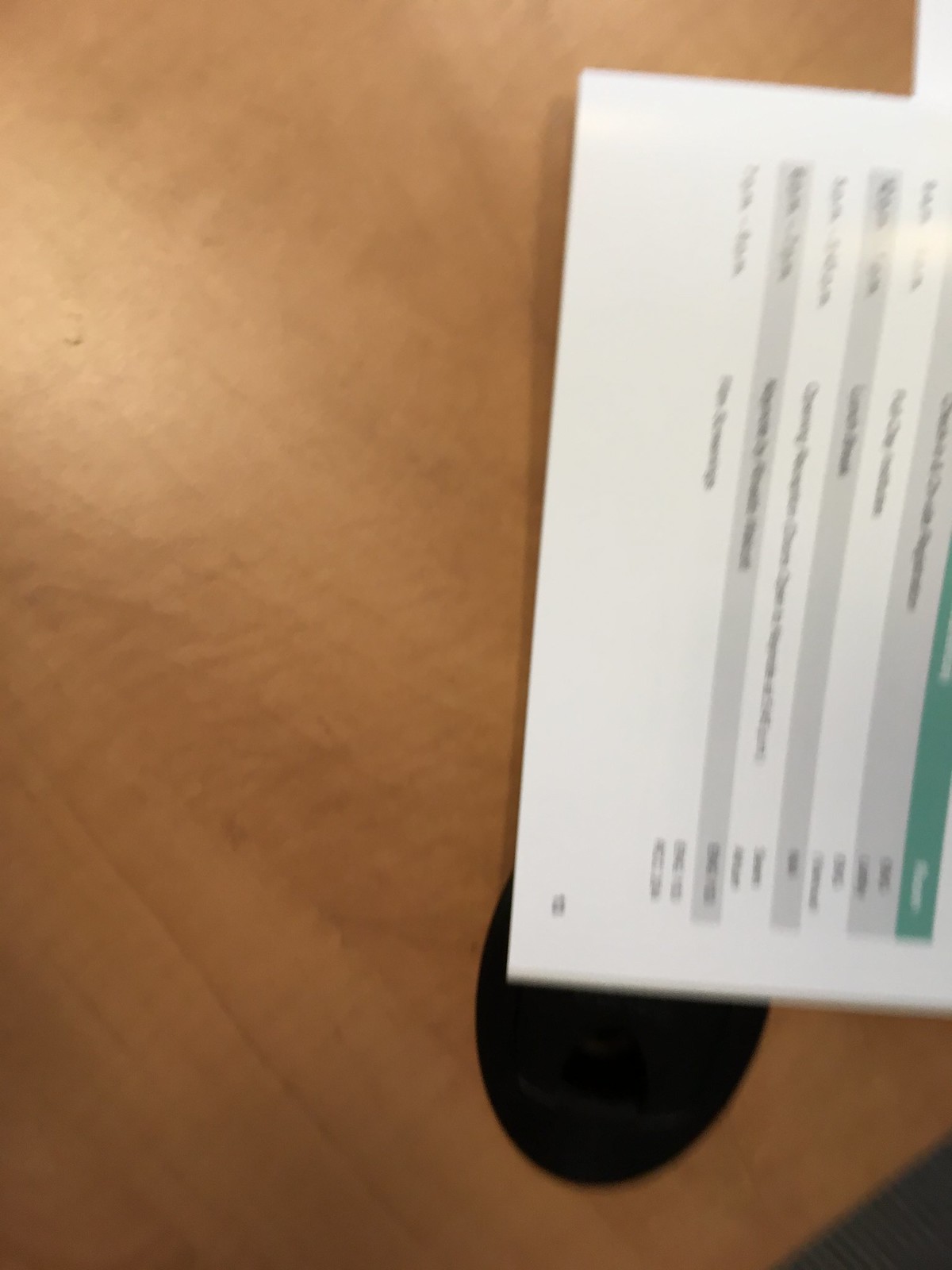A wood-toned desk sits against a backdrop of dark gray carpet flooring, suggesting an office environment. On the desk lies a partially visible, white sheet of paper featuring an informational table with gray and green lines. The content of the paper is blurry and unreadable, adding an element of mystery to the scene. Additionally, there seems to be a black object, possibly another desk or a chair, that is partially obscured by the paper, further adding to the intrigue of this office setting.